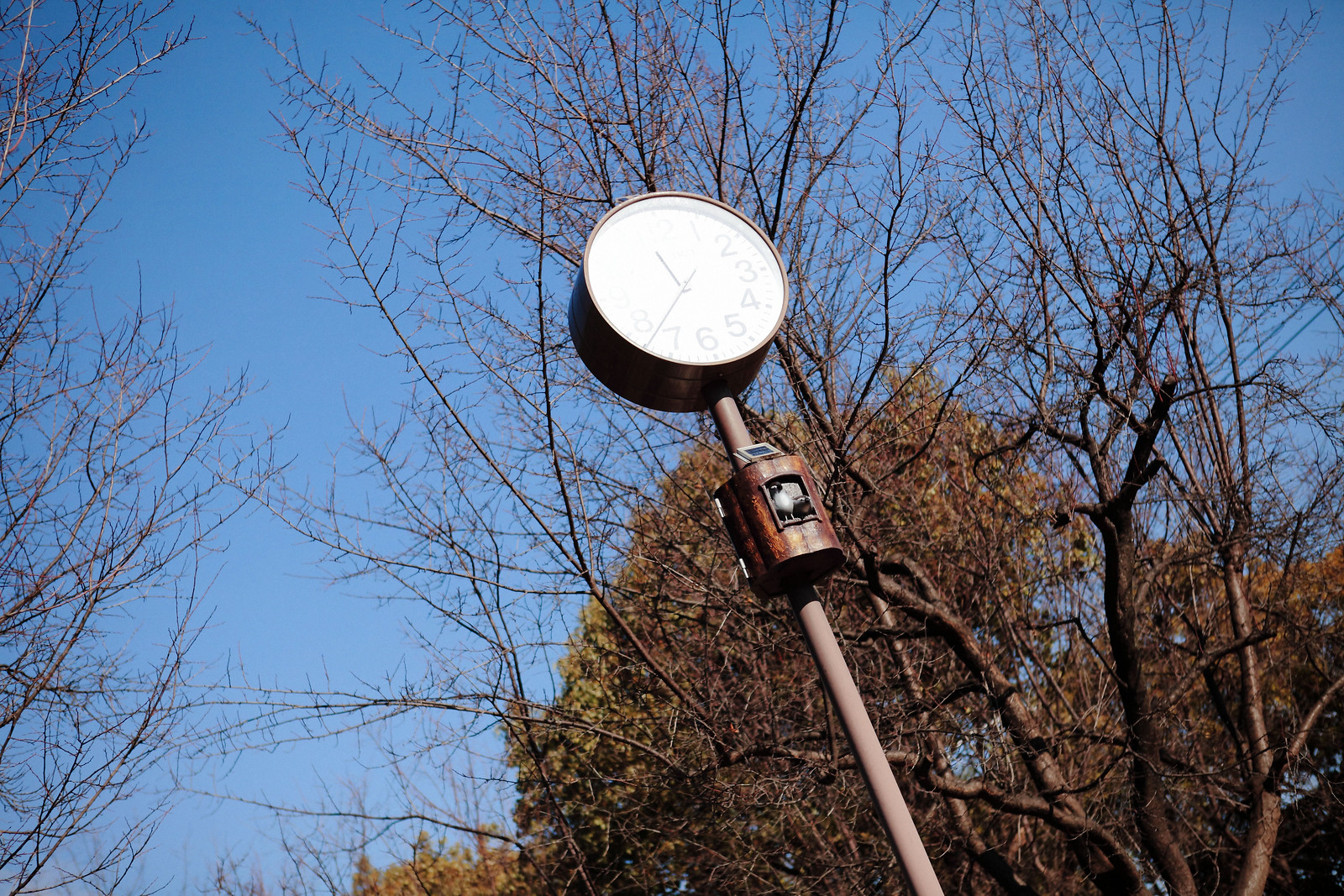The photograph captures a detailed and intriguing scene centered around a tall, copper-colored pole with a clock mounted on top. The clock, which has a thick bronze frame and a white face, features black numbers and hash marks, and currently displays the time as 11:38. There is a noticeable glare on the clock's face, likely reflecting the sun which is not visible in the frame. Directly beneath the clock is a small, bronze chimer, equipped with a gray solar panel on top and an open latch design. Perched within this chimer is a gray bird, with another bird standing next to it, both oriented to the right.

Surrounding the pole and clock is a picturesque natural background. The photograph, taken on a sunny day with a clear blue sky, shows a variety of trees at different stages of leaf development. In the foreground, the trees are mostly devoid of leaves, showcasing their bare branches, some of which have budding new growth. Further back, there is a mix of trees with leaves in varying shades of golden yellow, light green, and orange, painting an autumn-like tapestry against the blue sky. Unique branches, some broken and others extending in various directions, add character to the scene, along with the distant trees sporting red and yellow leaves, enhancing the photograph's depth and vibrancy.